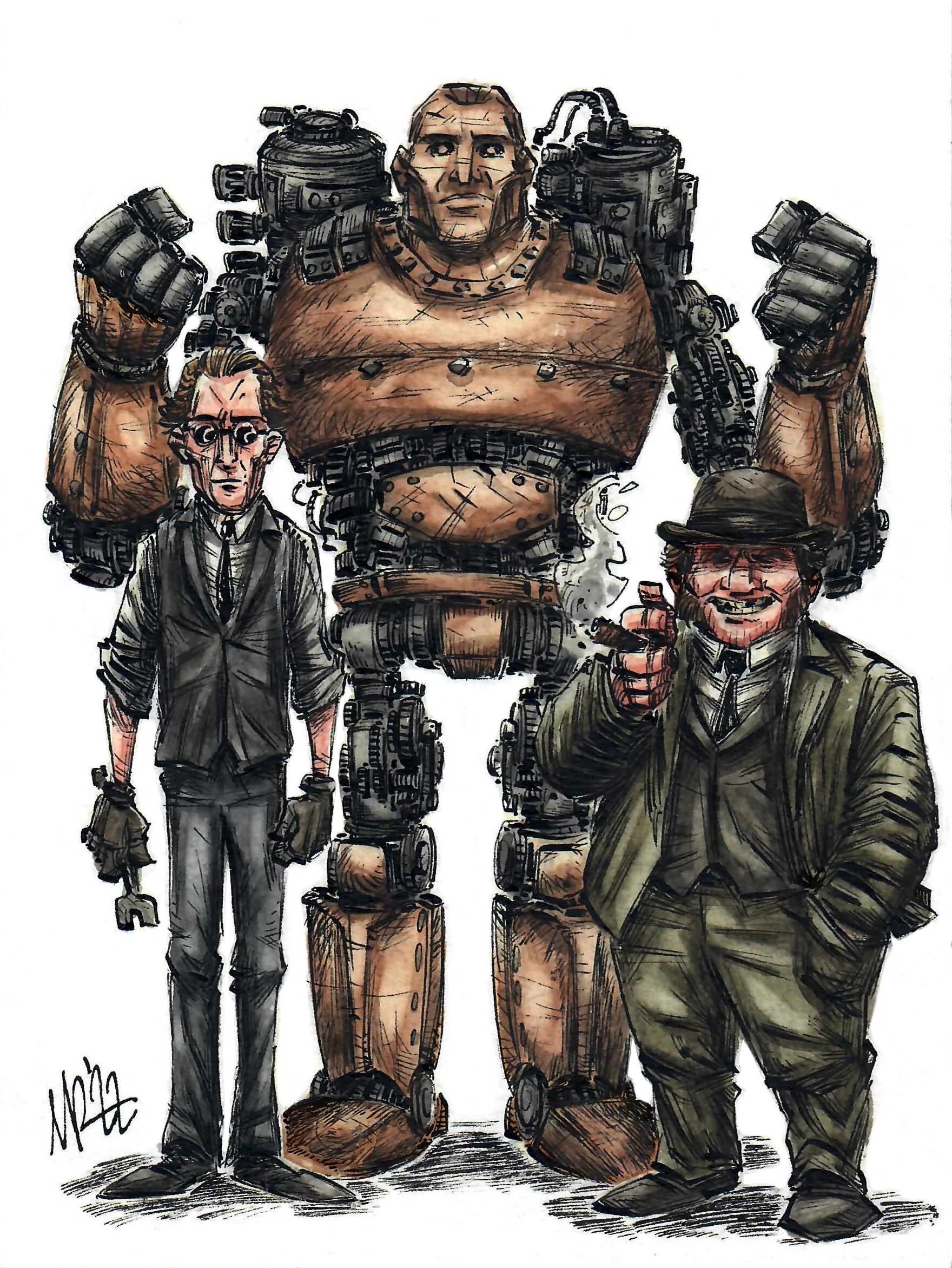In this detailed concept drawing, an artist's signature is located at the bottom left corner, indicating its hand-drawn nature. The composition features three distinct characters side by side: 

- On the left, there is a slim, bespectacled engineer, identifiable by his glasses or goggles and his attire, which consists of a white shirt, a vest, and a tie. He holds a wrench in his right hand, suggesting his role is mechanical or technical. He is also wearing work shoes and gloves indicative of his trade.
  
- The center figure is an imposing robot with a human head, characterized by a brown beard and vacant brown eyes. Its body is constructed from various mechanical parts, including a vest-like armor, powerful robotic arms, and legs adorned with gold boots. Two blaster-like components are mounted behind it, enhancing its futuristic appearance.

- On the right stands a short, stout man, depicted as a slimy investor or businessman. His appearance is marked by a suit, a gangster-style hat, and a cigarette in hand. He is the only one smiling in the image, adding a sinister aspect to his character.

Together, these figures create a multifaceted scene, blending elements of technology and human characteristics.